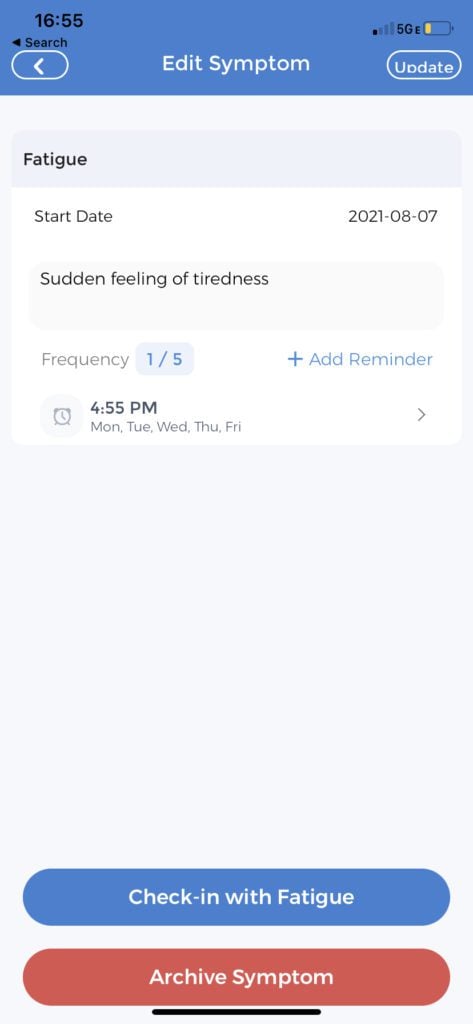This is a detailed caption for an image:
---
The image is a screenshot from a cell phone, prominently featuring a blue status bar at the top. In the top-left corner, the time is displayed as 16:55. The title "Edit Symptom" appears in white font within the blue bar. The device shows only one bar of cell phone reception on the upper right side, along with a 5GE network indicator. Adjacent to this, the battery icon is visible, indicating a 25% charge. Below the battery icon is an "Update" button.

On the far left of the blue status bar, there is a back arrow icon, which is a white arrow on a blue circular background with a white border. Moving down, the screen displays the current symptom being edited, titled "Fatigue." Beneath this, the start date is listed as "2021-08-07." The description, "a sudden feeling of tiredness," follows.

Further below, the frequency of the symptom is noted as "1 out of 5." At the bottom of the screen, there is a reminder set for 4:55 p.m. on weekdays: Monday, Tuesday, Wednesday, Thursday, and Friday.